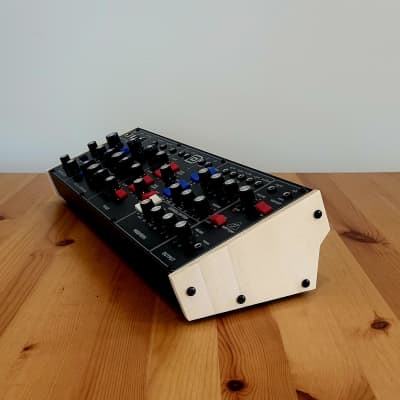The image features an older-style soundboard situated on a natural oak wood table, with its distinct wood grain and knots visible. The backdrop is a muted gray wall. The soundboard is long and rectangular, designed to be slightly angled with a higher back and lower front. It has a white side panel secured with four black screws. The top surface of the soundboard is predominantly black, adorned with numerous labeled knobs—black with white tops, silver, white, and blue. There are red and blue buttons interspersed among the knobs, along with switches on the right-hand side. The labels are in white text, and there's a logo at the top. The overall design indicates that the machine is likely used for managing audio recordings.